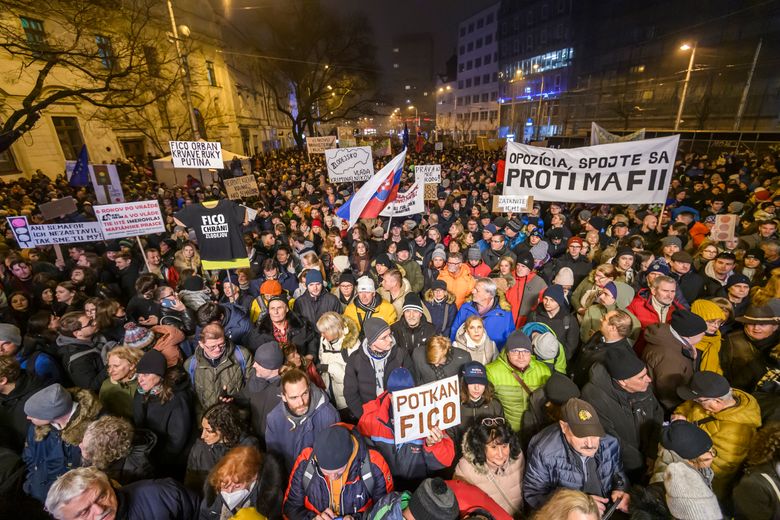This detailed photograph captures a nighttime protest in what appears to be Slovakia. The scene showcases a mass of demonstrators filling a wide city street. The sky above is completely dark, yet the area is well-illuminated by streetlights and possibly a spotlight, which highlights the central figures in the crowd while casting the edges into shadow.

The protesters, dressed in warm puffy jackets and a mix of baseball caps and ski hats, indicate a chilly evening. Both men and women are present, though women generally do not wear hats. The atmosphere, while determined, remains peaceful without any visible signs of misbehavior or agitation.

Many protesters carry signs, most of which are written in Slovak. Prominent among them are references to "FICO," likely pertaining to Robert FICO. Specific signs include phrases like P-O-T-K-A-N F-I-C-O and a longer message reading O-P-O-Z-I-C-I-A, S-P-O-J-T-E S-A P-R-O-T-I M-A-F-I-I. The lined street is flanked by buildings, some of which have lights on, adding depth to the urban night scene. This organized, peaceful demonstration reflects a collective resolve, standing out against the backdrop of the Slovak city’s illuminated architecture.